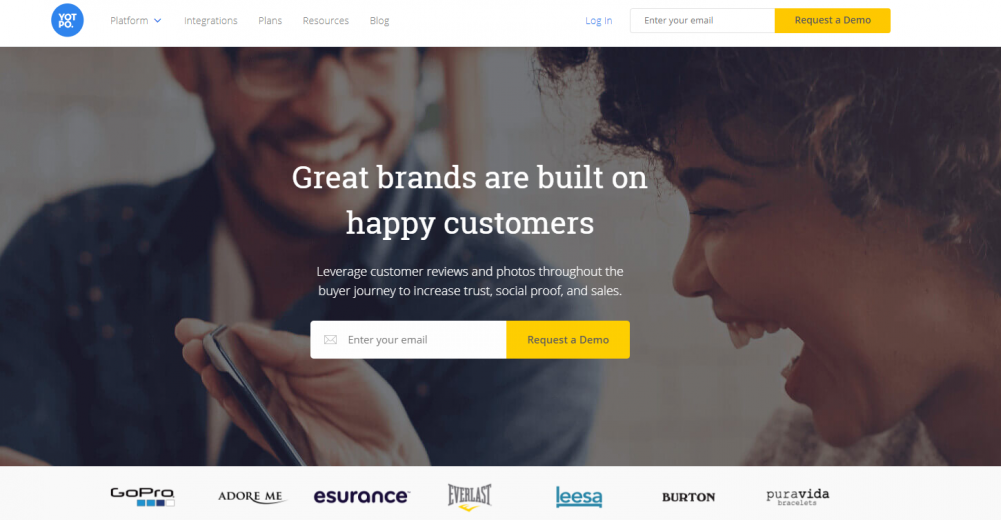On a clean white background, a polished webpage is prominently centered, featuring a vivid blue circle on the left side. Within this circle, the words "Vote PO" are displayed. Adjacent to the circle, in grey text, there's a navigation bar that lists "Platform," "Interrogations," "Plans," "Resources," and "Blog." Towards the far right of the navigation bar, there is a "Login" button. Below this, you can find an input field prompting users to enter their email address, followed by a striking "Request a Demo" button in yellow text against a black background.

The central portion of the page features a heartwarming image of two people laughing exuberantly. The woman, who is on the right-hand side, is glancing at her smartphone while the man, positioned more to the left, looks at her with amusement. Overlaying this image, white text reads: "Great brands are built on happy customers. Publish customer reviews and photos through the buyer journey to increase trust, social proof, and sales."

Directly below this are additional fields for users to enter their email and another prominent "Request a Demo" button, emphasizing their strong call to action.

At the very bottom of the page, various brand logos are showcased, including recognizable names such as GoPro, Adobe, Meet, Ensure, Everlast, Elisa, Burton, and Pure Vita.

The scene transitions unexpectedly to a stairwell, where a woman is seen ascending, leading to the imagery of an upward journey. This is evocative of the classic theme of moving up to a better place, symbolizing growth and progress.